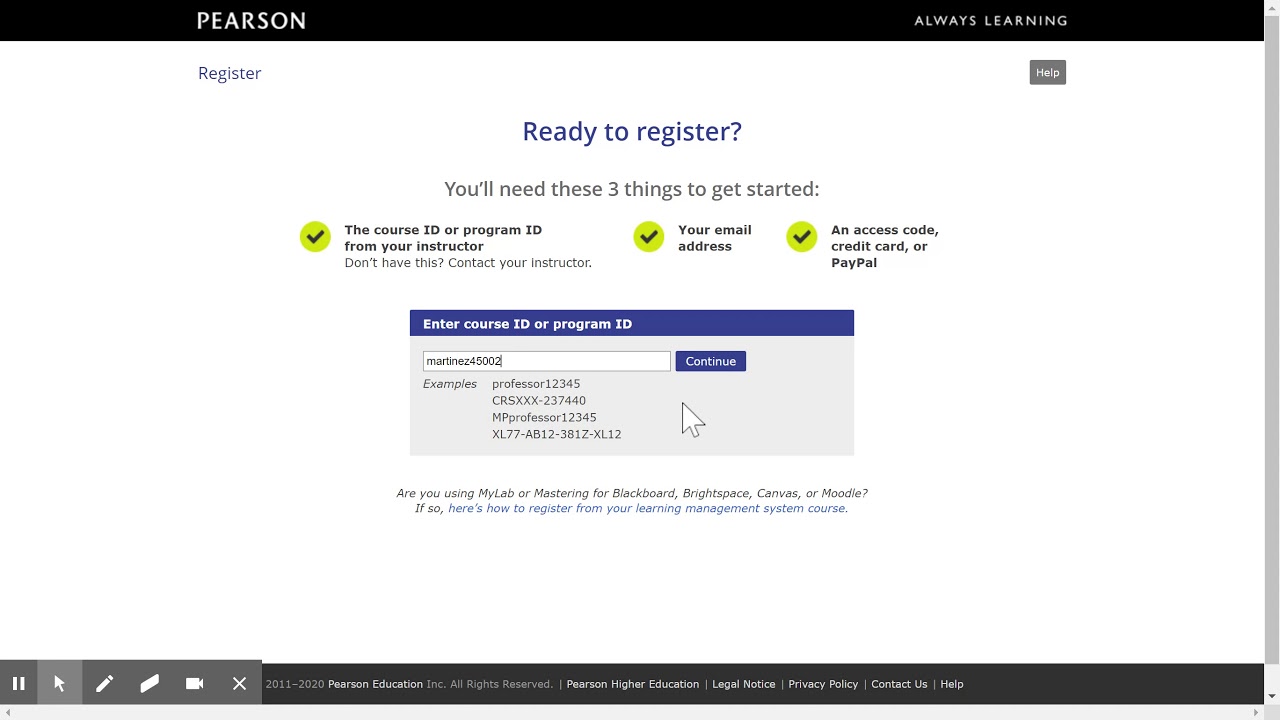The Pearson website features a sleek, modern design with a black banner across the top. Positioned approximately one-quarter of the way from the left is the Pearson logo, subtly balanced by their motto, "Always Learning," on the opposite side of the banner. Directly beneath this, a large white screen dominates the page, offering a clean, minimalist look.

At the top of the white screen, just below the Pearson logo, small gray text provides navigational options: "Register" on the left and "Help" on the far right. Centrally aligned in a medium blue font is the question, "Ready to register?" A couple of lines below, in gray text, reads the prompt: "You'll need these 3 things to get started," followed by a checklist.

The checklist consists of three essential items, each accompanied by a green disc highlighted with a blue check mark:
1. **Course ID or Program ID from your instructor** – If you're missing this, a clickable notice directs you to contact your instructor.
2. **Your email address.**
3. **An access code, credit card, or PayPal.**

Below the checklist, there is an input field where you can enter your Course ID or Program Number, along with a ‘Continue’ button to proceed. This intuitive layout ensures that users can smoothly begin their educational journey with Pearson.